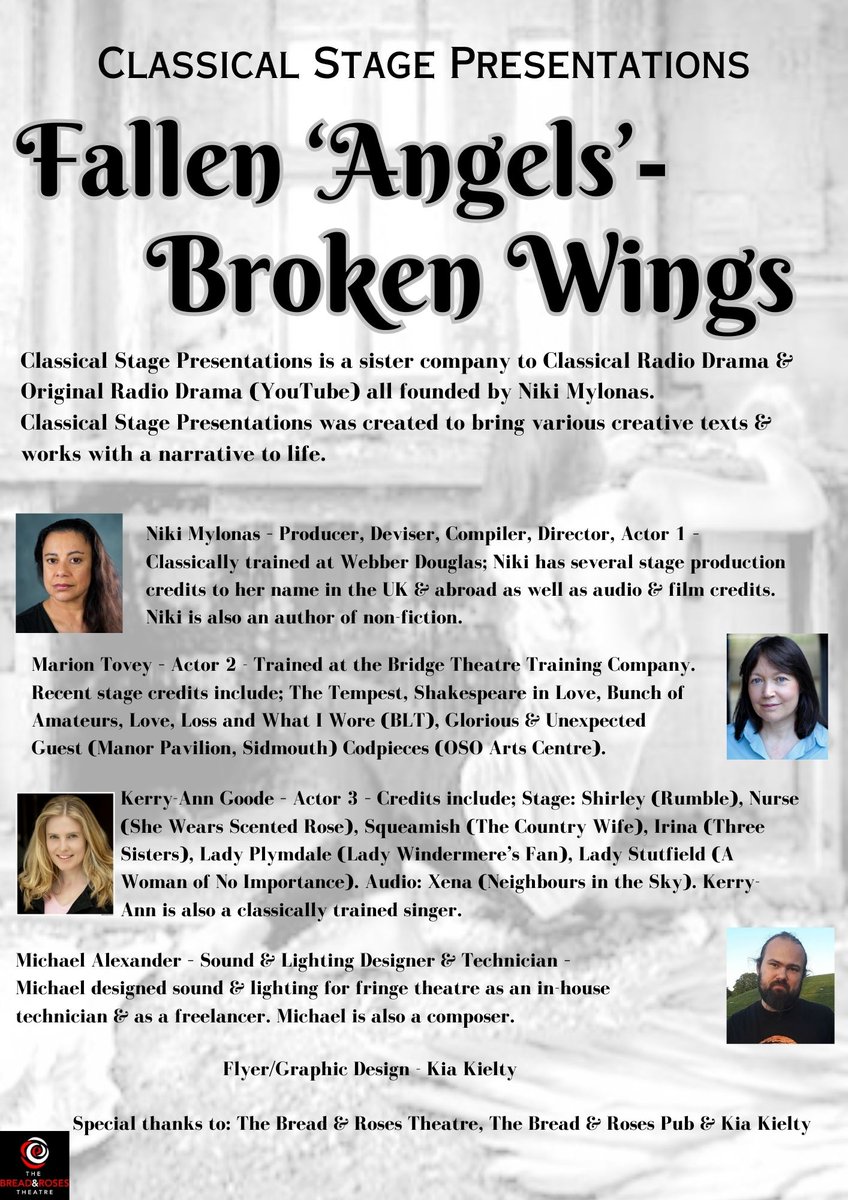This black-and-white flyer, promoting a theatrical drama, features a detailed title at the top, "Classical Stage Presentations" in bold black text, followed by "Fallen Angels, Broken Wings" in an elegant, flowy script outlined in light gray. The flyer provides an overview of Classical Stage Presentations, a sister company to Classical Radio Drama and Original Radio Drama on YouTube, all founded by Nikki Milonis. The company's mission is to bring various creative texts and narrative works to life. 

The central portion of the flyer highlights profiles of key team members with their photos and brief bios: 

- **Nikki Milonis**, a woman with long brown hair wearing a black shirt, is introduced as the Producer, Devisor, Compiler, Director, and Actor One. Trained at Weber Douglas, she is credited with multiple stage productions in the UK and abroad, along with audio and film endeavors. Nikki is also a non-fiction author.
  
- **Marion Tovey**, with black hair, is Actor Two. Trained at the Bridge Theatre Training Company, her recent stage performances include "The Tempest," "Shakespeare in Love," "A Bunch of Amateurs," and others.
  
- **Carrie Ann Good**, a blonde woman in a black and pink shirt, is Actor Three. Her stage credits include "Shirley Rumble," "Nurse She Wears Scented Roses," and "Lady Windermere’s Fan." She is a classically trained singer with several audio credits, including "Xena" and "Neighbors in the Sky."
  
- **Michael Alexander**, depicted with a brown beard and wearing a black shirt, is the Sound and Lighting Designer and Technician. Michael’s work spans fringe theater and freelance projects as well as composing music.

Also credited on the flyer are special thanks to The Bread and Roses Theatre, The Bread and Roses Pub, and Kia Keltley for flyer/graphic design. The background image displays a vague figure of a woman, adding a mysterious touch to the overall design.